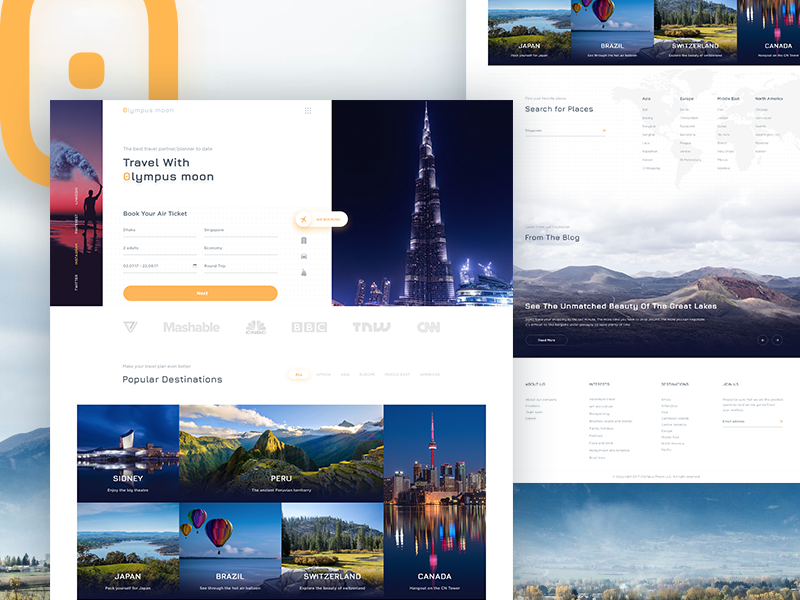The collage in the image is a vibrant and dynamic travel-themed montage bursting with inspiring destinations and travel-related information. 

In the upper left corner, bold text reads "Travel with Olympus Moon," accompanied by a prompt to "Book Your Air Ticket." Adjacent to this text is a captivating night-time photo of an impossibly tall building, tapering off into a spire, glowing against the darkness. To the left of this, an evocative image captures a person silhouetted against a breathtaking sunset, holding an item that emits colorful smoke.

Below these is a headline that declares "Popular Destinations," under which sits an array of photographs showcasing global landmarks. Each photo is meticulously labeled: one depicts the iconic Sydney with its stunning coastline, another captures the rugged beauty of mountains in Peru. A serene lake nestled within a rural setting is labeled Japan, while vibrant hot air balloons hover over water in Brazil. A dense, lush forest represents Switzerland, and a reflective cityscape shimmering against a body of water signifies Canada. 

On the left side of the montage, smaller versions of some of the previously mentioned images appear, anchored by a search box under the heading "Search for Places." Below this, a blog promotion reads "From the Blog," superimposed on a dramatic outdoor photo with a cloudy sky, mountains, and rolling hills, inviting viewers to "See the Unmatched Beauty of the Great Lakes."

At the bottom of the image, blurry text hints at additional information about the site. The visual narrative is tied together with a final image featuring an expansive sky bursting with twilight hues above a silhouetted forest of trees.

This meticulously arranged collage not only provides travel information but also teases the beauty and allure of global exploration.